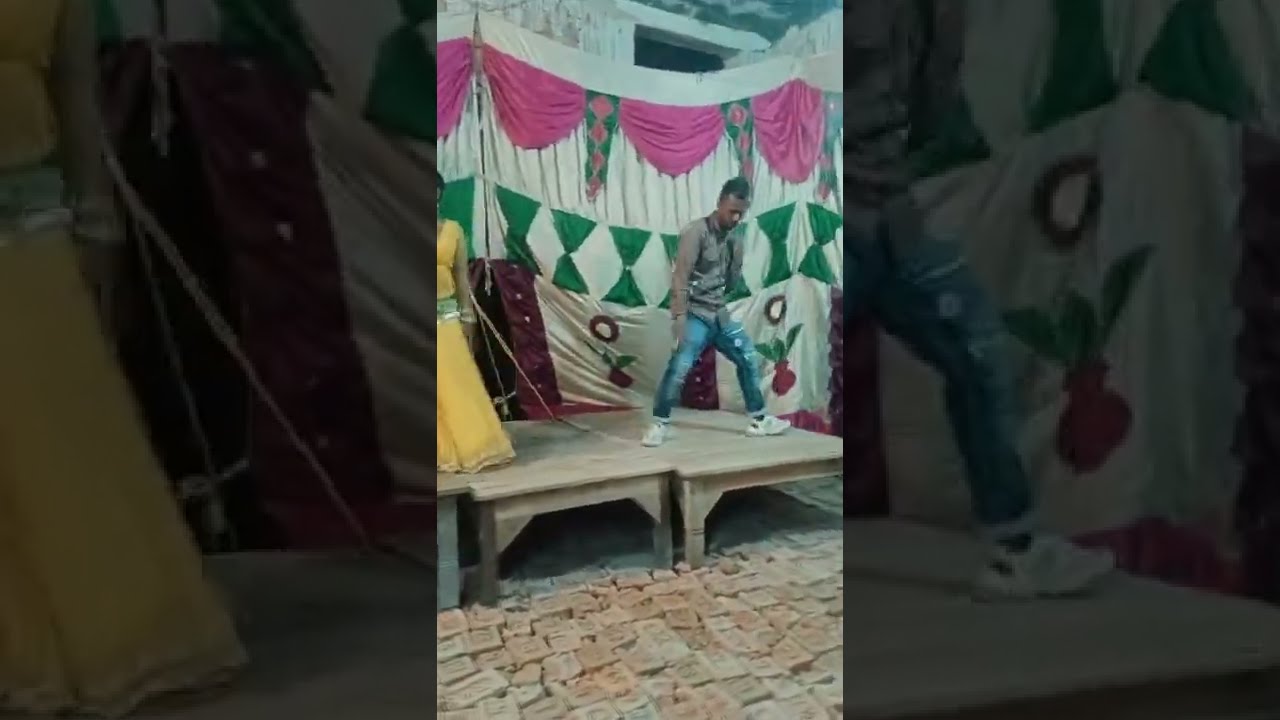In this photograph, a man stands on top of a makeshift stage composed of two adjacent wooden tables painted white, set on a worn, irregular cobblestone floor. He is dressed in a long-sleeved gray sweatshirt, denim jeans, and white sneakers, looking down towards his feet. The stage is flanked by a large, partially visible yellow curtain on the left, and behind the man hangs a prominent white curtain adorned with a purple valance at the top, green and pink flags, green triangles, and red circles with green leaves emerging from red bases. To the man's right, partially visible, stands a woman dressed in a long, sleeveless yellow dress or pantsuit. The photograph has shaded left and right thirds, highlighting the central scene.